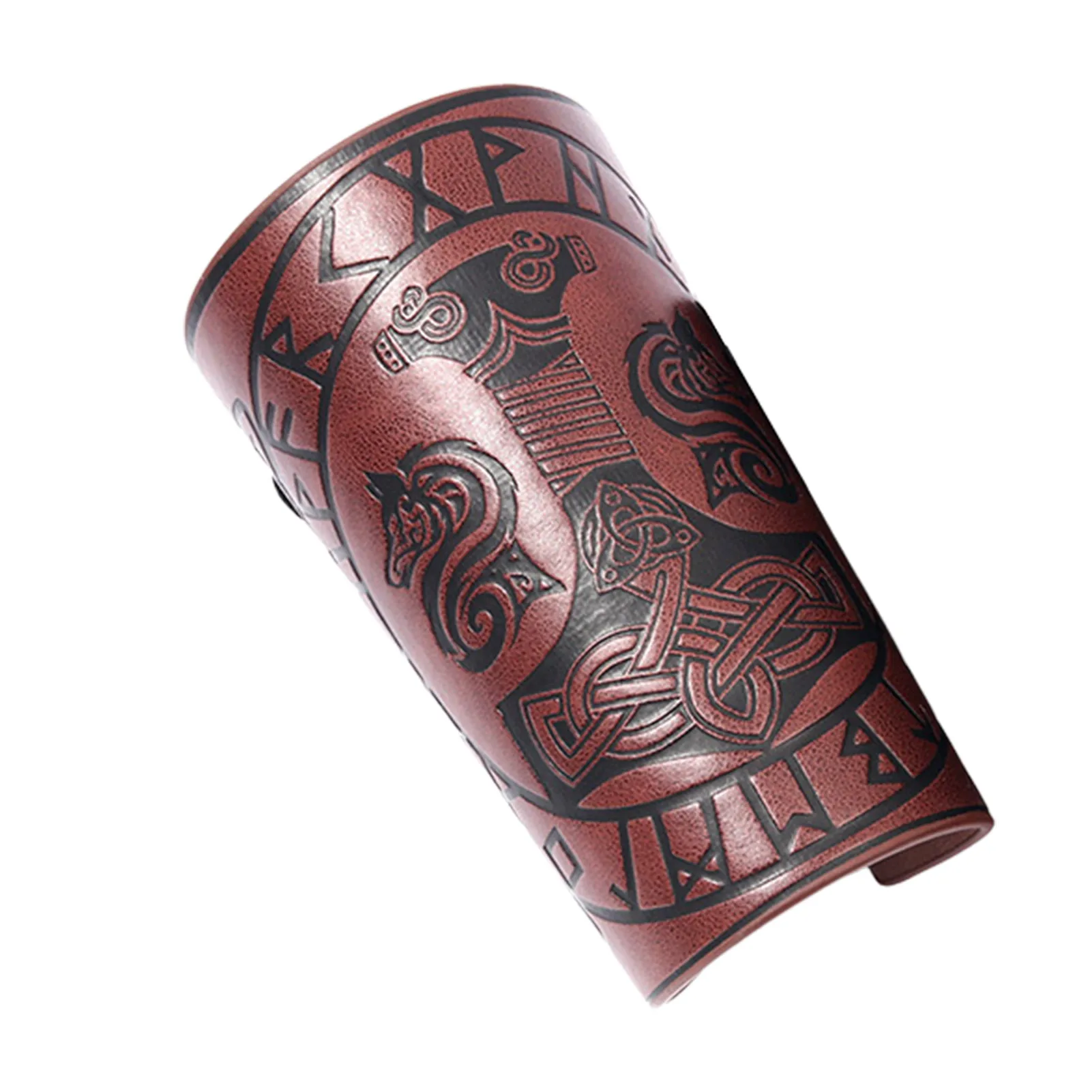The object in the photograph appears to be a leather armband or armlet, made from a reddish-brown leather material. The band is slightly curved, suggesting it would fit comfortably around a person's wrist to forearm, narrowing at the bottom and widening at the top. The armband is adorned with intricate black designs and symbolic markings. In the center, surrounded by a ring of runic or rune-like letters, are two stylized animal heads, which could represent dragons or wolves due to their broad, logo-like features. Between the animals, a hammer with a Celtic knot pattern—or possibly the handle of a sword with crisscrossed leather binding—is prominently featured. The detailed artwork, including interconnected lines and symbols, evokes a blend of Greek, Viking, or Celtic motifs. The object is presented against a stark white background, highlighting these elaborate details and ensuring no other distractions are present in the photograph.